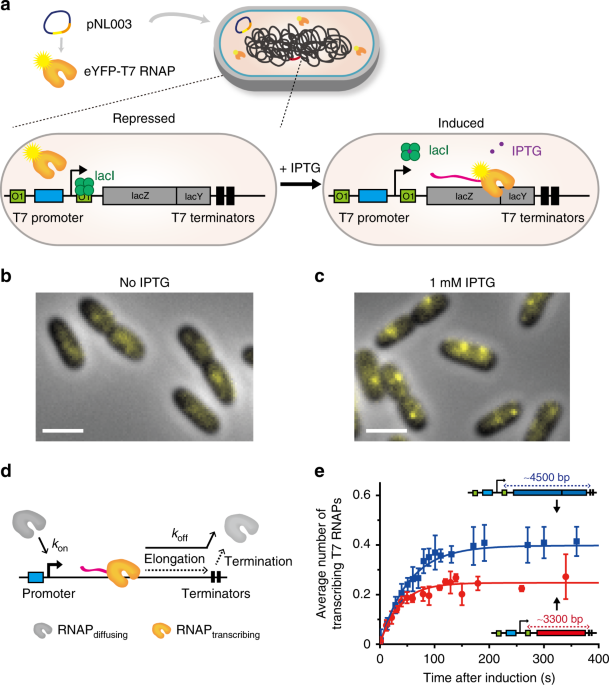The scientific graphic elucidates the progression from Step A to Step E, capturing detailed visual representations at each stage. At the top, Step A showcases a capsule-shaped diagram with a gray outer border and a light peach-colored interior, highlighting black squiggly lines and orange usage letters at the core. This section also features text labels indicating "PNL 003 eYFP-T7 RNAP" and "repressed," with additional elements such as T7 terminators and T7 promoters encapsulated within a gray rectangle centered by black outlines.

Moving down, Step B and Step C present images of microorganisms, each annotated as "no IPTG" and "1 mM IPTG" respectively. These two images are flanked by gray backgrounds and contain green and black shapes symbolizing cellular structures.

Further below, Steps D and E transition to graphical data. Step D includes a diagram illustrating RNAP diffusing through the cell, followed by RNAP transcribing. Step E presents a graph plotting the time of induction against the average number of transcribing RNAs, marked with red and blue data points and lines on X and Y axes. Collectively, the graphic uses a consistent color scheme of gray, cream, orange, green, blue, yellow, and black to convey intricate scientific processes and data correlations.